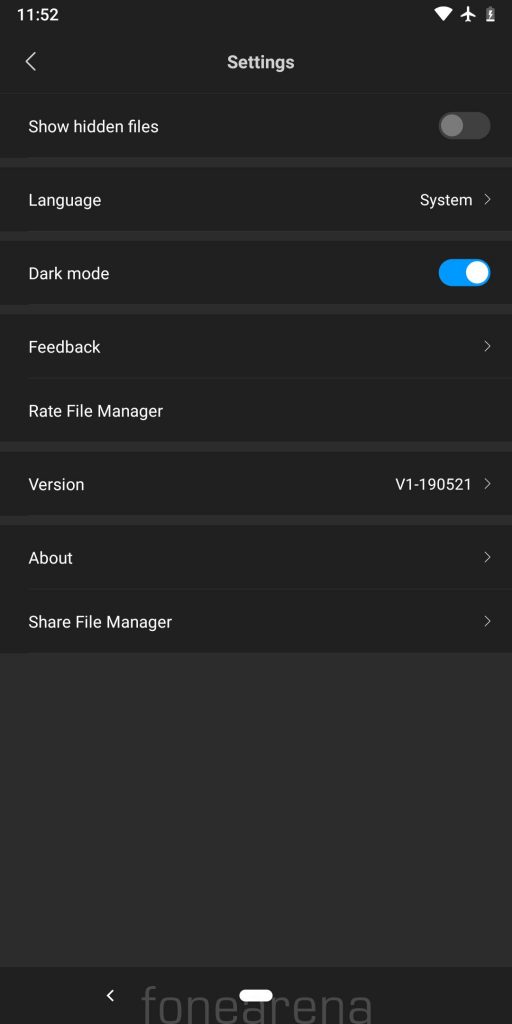The image depicts a mobile or tablet interface on a website, featuring a predominantly black background with white text. In the upper left-hand corner, the number "1152" is visible, while icons for Wi-Fi, airplane mode, and another unclear icon are present in the upper right-hand corner, suggesting it might be on airplane mode. 

Central to the image is a settings menu with a back arrow on the left. Below that, the option "Show Hidden Files" is listed with a toggle slider that is off. Thin grey horizontal lines separate these menu items for clear delineation. The menu includes options such as "Language" with "System" noted on the right, "Dark Mode" with an active blue slider, and "Feedback". The list continues with "File Manager", "Rate File Manager", and a version number "wi-190521" to the right. Further down, "About" includes right-pointing arrows for navigation, followed by "Share File Manager".

At the bottom of the interface, a narrow white line is noted, with a central back arrow. There's also a dark band, potentially a watermark, with partially visible text possibly indicating "Phone Arena". This suggests the screenshot might have been taken from a webpage or app interface displayed on a mobile or tablet device.